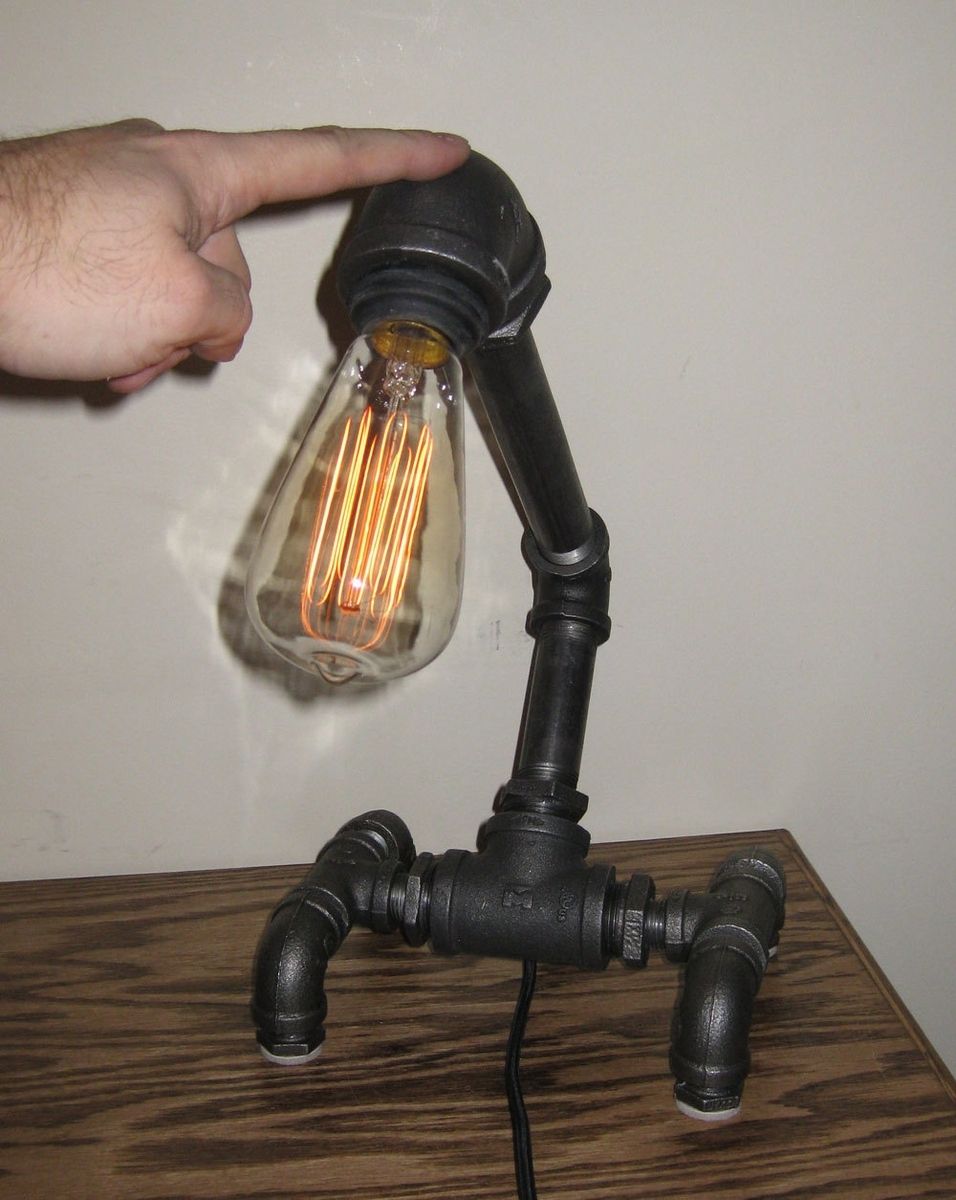The photograph features an intricately designed desk lamp seated on a pale brown wooden desktop with dark brown grain patterns. The lamp is crafted from black cast iron plumbing pipes, meticulously jointed together to form a structure with a sturdy double stand and a long, elegant neck leading up to the bulb. The bulb itself is a striking feature, shaped like an elongated vase—wider at the bottom and tapering towards the top. It houses a series of thick, curved filaments arranged in a circular pattern, which glow brilliantly in hues of orange and red. A black cord extends from the center of the lamp, and the entire setup is set against a plain white wall. Captured in the image is a man's left hand, noticeably hairy up to the wrist, gently touching the top of the lamp with the fingertip.